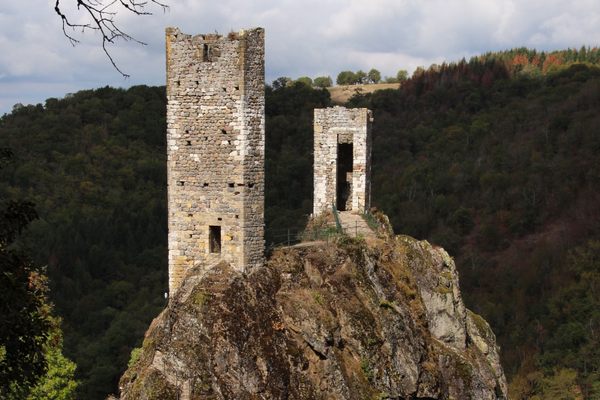The image captures the serene and historical beauty of a ruined medieval castle perched on a rocky, treeless hill amid a striking mountainscape. Central to the scene are two tall, crumbling stone towers, constructed from grey and beige cobblestone bricks. These ancient towers are connected by a small fenced walkway, indicating recent efforts to preserve and possibly allow access to the site. The fence appears green, contrasting with the rugged stone of the towers. Beyond this rocky outcrop, the background reveals a lush mountain range dotted with green trees and colored foliage, suggesting a fall setting. The sky above is a mix of blue with patches of fluffy clouds, adding depth to the tranquil landscape. In the top left corner, some leafless tree branches droop into the frame, hinting at the seasonal change or the presence of an unkempt or dead tree nearby.